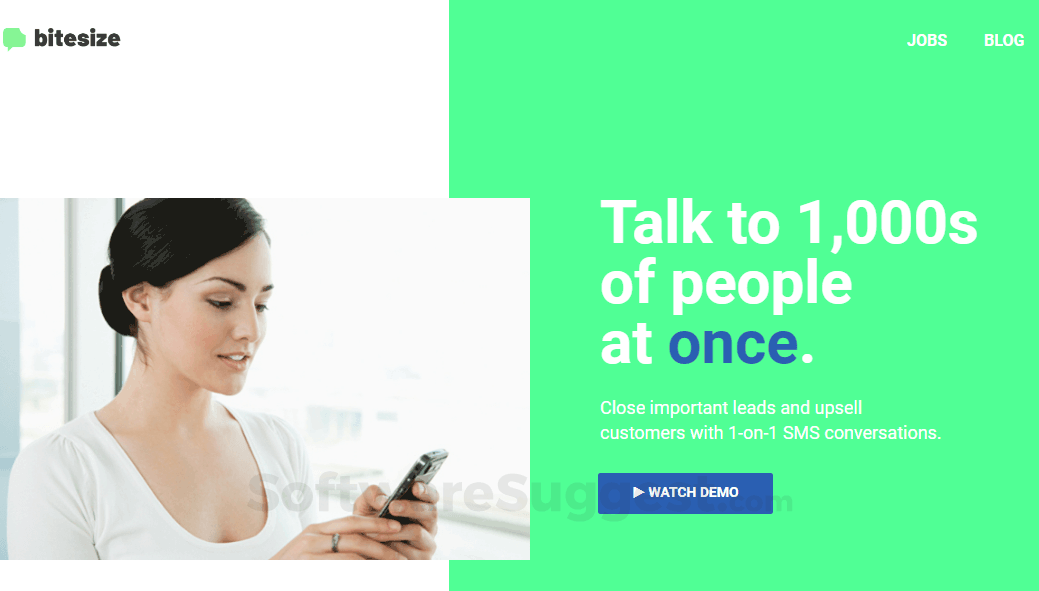The screenshot captures the homepage of the ByteSize website. The top-left corner prominently displays the ByteSize logo, consisting of bold, lowercase black text accompanied by a green brain-like icon. Below the logo, an image features a woman holding her phone with both hands, her head tilted down as she focuses intently on the screen, possibly spelling out or saying something. She has short black hair tied in a ponytail and is dressed in a low-cut, white shirt. The background on the left side of the screenshot is white.

On the right side, the background transitions to green. At the top-right corner, two tabs labeled "Jobs" and "Blog" are visible, inviting users to explore different sections of the website. Below these tabs, a large white text phrase commands attention: "Talk to thousands of people at once." Underneath, a secondary text line reads, "Close important leads and upsell customers with one-on-one SMS conversations," highlighting the website's offerings.